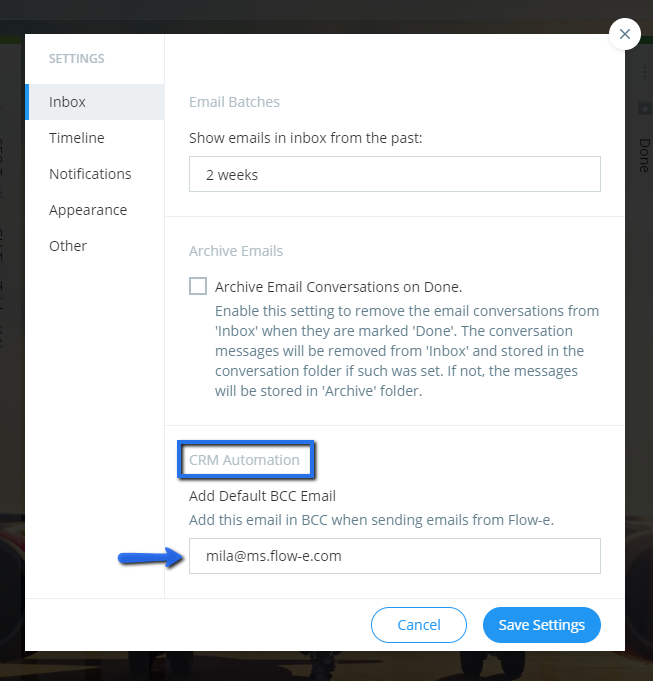The depicted image showcases the inbox settings menu within a settings page, set against a predominantly blackish background featuring a faint, indiscernible image. In the foreground, a white settings window stands out. 

On the left side, a vertical menu lists various options, with the header "Settings." Below this header, the following options are listed: "Inbox," "Timeline," "Notifications," "Appearance," and "Other," with the "Inbox" option highlighted, indicating it is currently selected.

To the right of this menu, a larger box presents detailed inbox settings. At the top of this box, the title "Email Batches" is displayed. Directly underneath, it reads, "Show emails in inbox from the past," accompanied by a dialog box displaying "Two weeks," indicating a selection to display emails from the past two weeks.

The subsequent setting is "Archive Emails," followed by a checkbox labeled "Archive email conversations on done," which appears to be an actionable option.

The third setting, "CRM Automation," outlined in blue, includes the instruction "Add default BCC email." The corresponding dialog box contains the email address "Mila@MS.flow.e.com," highlighted by a blue arrow pointing towards it.

At the lower right corner of the settings window, there are two buttons: one labeled "Cancel" and the other "Save Settings," the latter in blue, signaling it as the primary action button.